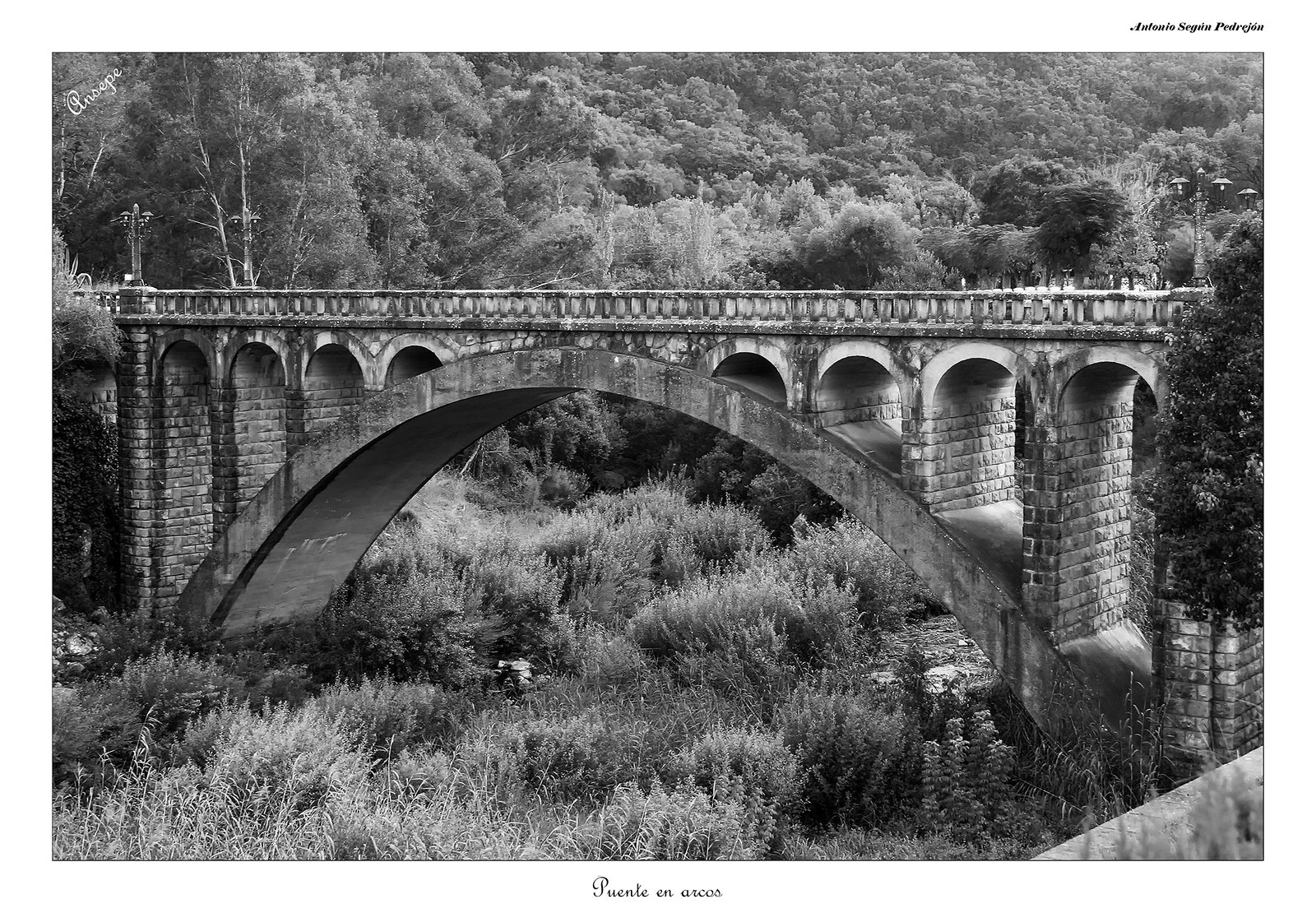This is a detailed black and white photograph of a historic stone bridge stretching from the left to the right side of the image. The bridge features a prominent large arch in the center, flanked by four smaller arches on either side. At the top, the bridge is flat, and along its sides, there are light posts, possibly with two to four lights each. Below the bridge, overgrown bushes or grass are present, with a small river or creek flowing underneath. In the background, a dense canopy of trees creates a natural backdrop, adding to the photograph's timeless and serene atmosphere.